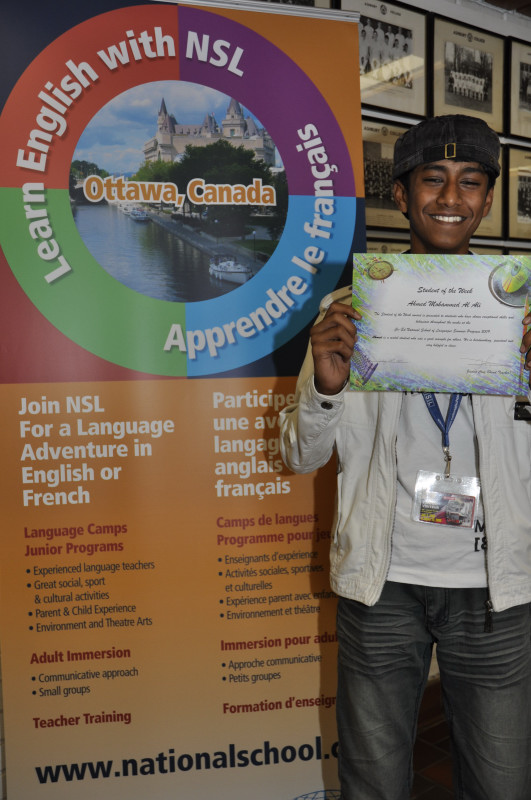A young, dark-skinned boy with dark hair stands proudly in front of a vibrant, multicolored sign, holding a certificate close to his chest. He is wearing a white jacket over a white t-shirt, blue jeans, and a blue lanyard with laminated identification hanging from it, and he has a black baseball cap turned backward on his head. The sign to his right is prominently displayed and reads "Learn English with NSL" at the top, with "Ottawa, Canada" in the center, along with a scenic picture of a river with boats and a castle. Below, it encourages joining NSL for a language adventure in English or French, with text also provided in French: "Apprendre le Français." The background includes a wall adorned with numerous black-and-white photos in black frames. The certificate the boy holds appears to recognize his achievement, possibly stating "Student of the Month" amid various shapes and text, though the exact wording is hard to discern. At the bottom of the poster, the NSL school website, www.nationalschool.com, is listed.